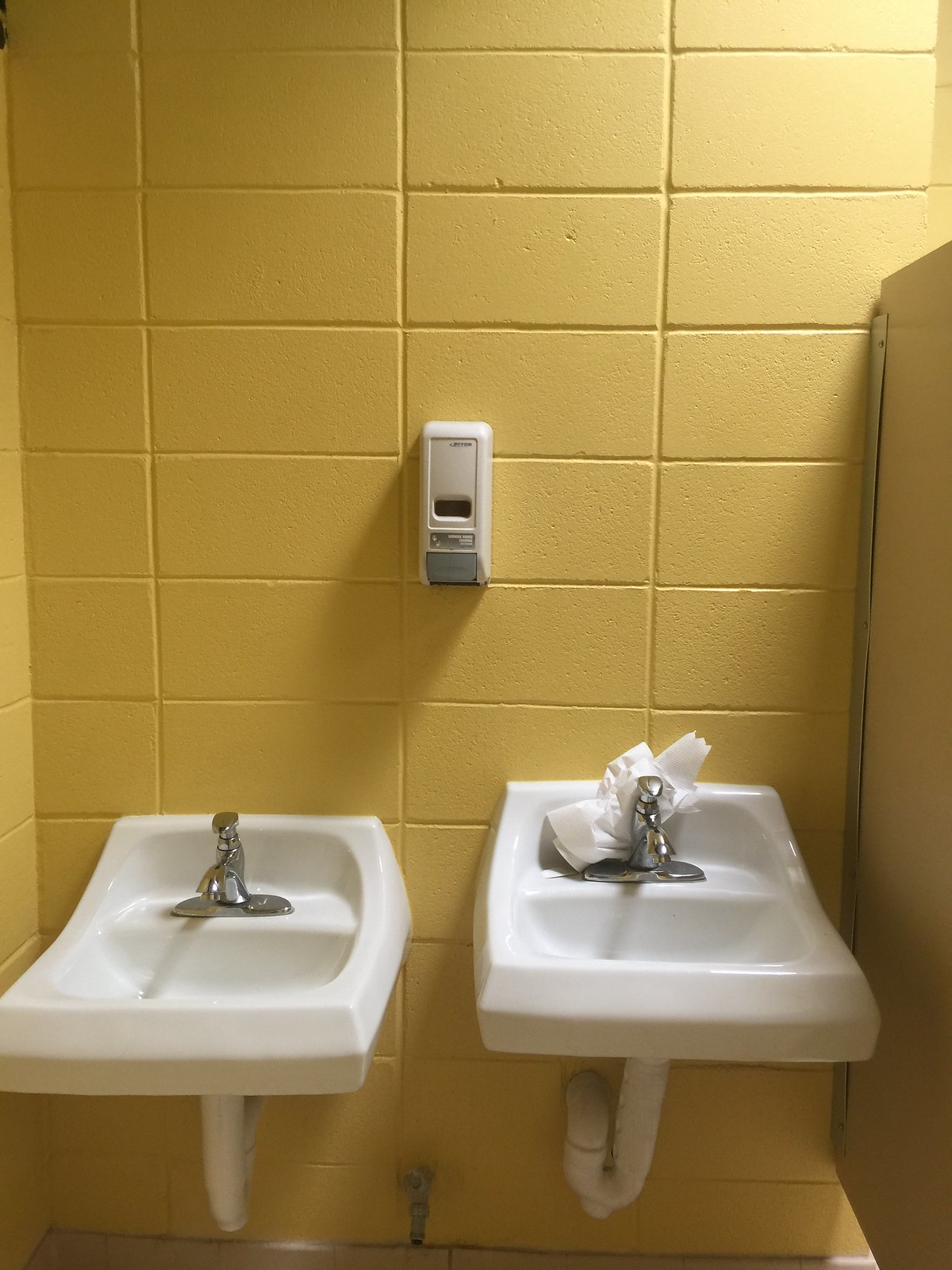This is a photograph of an interior public bathroom, potentially in a school or government building, characterized by its generic, utilitarian design. The back wall is composed of yellow-painted cement blocks, arranged in a grid-like fashion. Prominently displayed between two porcelain sinks is a white, off-colored soap dispenser with a grey push panel and a small, dark grey window for viewing the soap level. On the left side of the image, a lower sink features a silver faucet and white drainage pipes underneath. To the right, a slightly higher sink—raised by about two or three inches—also has a silver faucet and white piping, with a piece of white paper towel bunched up behind it. The right side of the image also shows a greyish partition wall that likely forms part of a toilet stall. Both sinks are mounted directly to the wall without any countertop space, underscoring the basic functionality of the setting. There is a small, silver spigot located at the bottom center of the image, emerging from the wall.